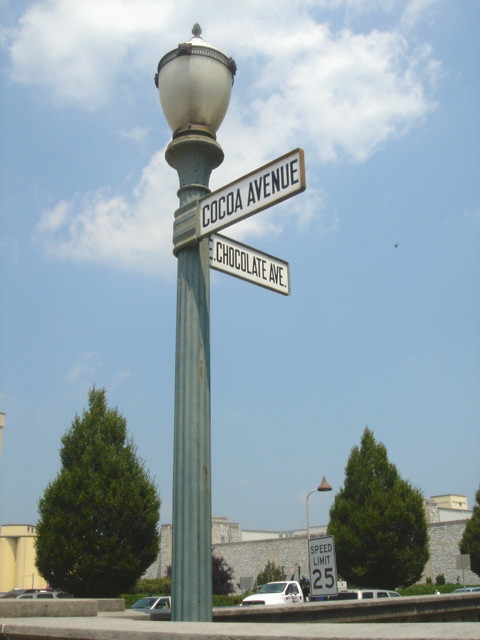The image depicts a downtown street corner featuring a striking light post adorned with two white, black-lettered directional signs indicating Cocoa Avenue and East Chocolate Avenue, both named after candies. The light post, which is gray and topped with a large white globe encasing a lamp, stands prominently amidst a beautifully clear, bright blue sky dotted with small white clouds. Below the street signs, there is a speed limit sign marking 25 mph. Surrounding the street corner, the scene includes two large, green trees resembling Christmas trees. Vehicles, including a white truck and a partially seen silver truck, navigate East Chocolate Avenue as they pass by the trees. In the background, there are various buildings, including a white concrete structure and a smaller, beige one, adding to the urban landscape.